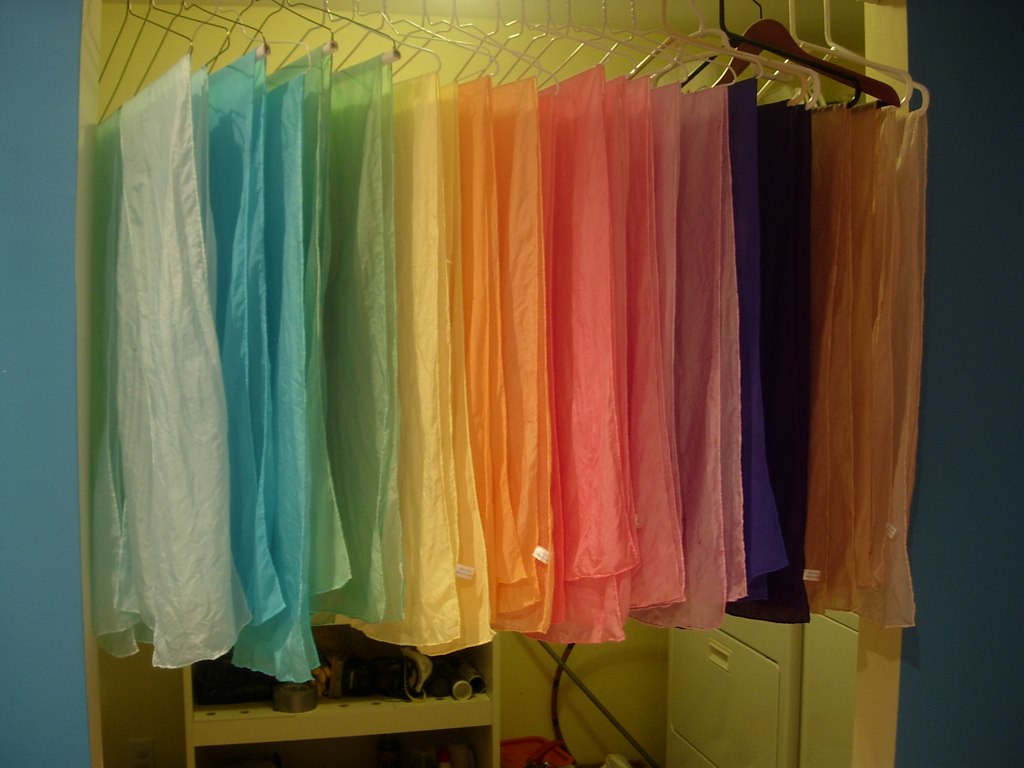The photograph showcases a vibrant assortment of sheer, rainbow-colored chiffon scarves hanging neatly on a clothes rack, which appears to mark the entrance to a laundry room. The scarves, which range in color from light blue, green, yellow, orange, pink, purple, dark blue, to a golden brown, are suspended from various types of hangers including metal, plastic, and wood. The backdrop consists of a sky-blue wall with an open doorway revealing a room lit warmly, casting a yellowish hue that makes the washing machine and dryer appear yellow, although they might actually be white. Inside the room, a yellow-walled background frames a bookcase stocked with duct tape and miscellaneous items, situated beside black wires trailing between the shelves and the dryer. Below the scarves, additional shelves and drawers can be seen, contributing to the organized appearance of the space.